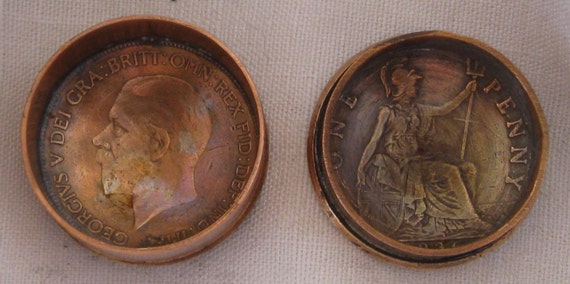The image showcases a close-up of two well-worn, bronze coins resting on a light cream Hessian-style tablecloth. The coin on the left features a side profile of a bearded man, likely King George, with Latin text, including "Brit" and "Rex," encircling his head. This coin is securely held within a raised, bronze holder. The coin on the right, labeled "ONE PENNY" in capital letters, depicts a woman in a wheelchair. She is dressed in a long robe and a Roman-style helmet, holding a trident in her left hand. This coin appears more greenish in hue compared to the other and is also seated in a similar bronze holder. Both coins have a distinctly antique and uneven surface, suggesting significant age and historical value.